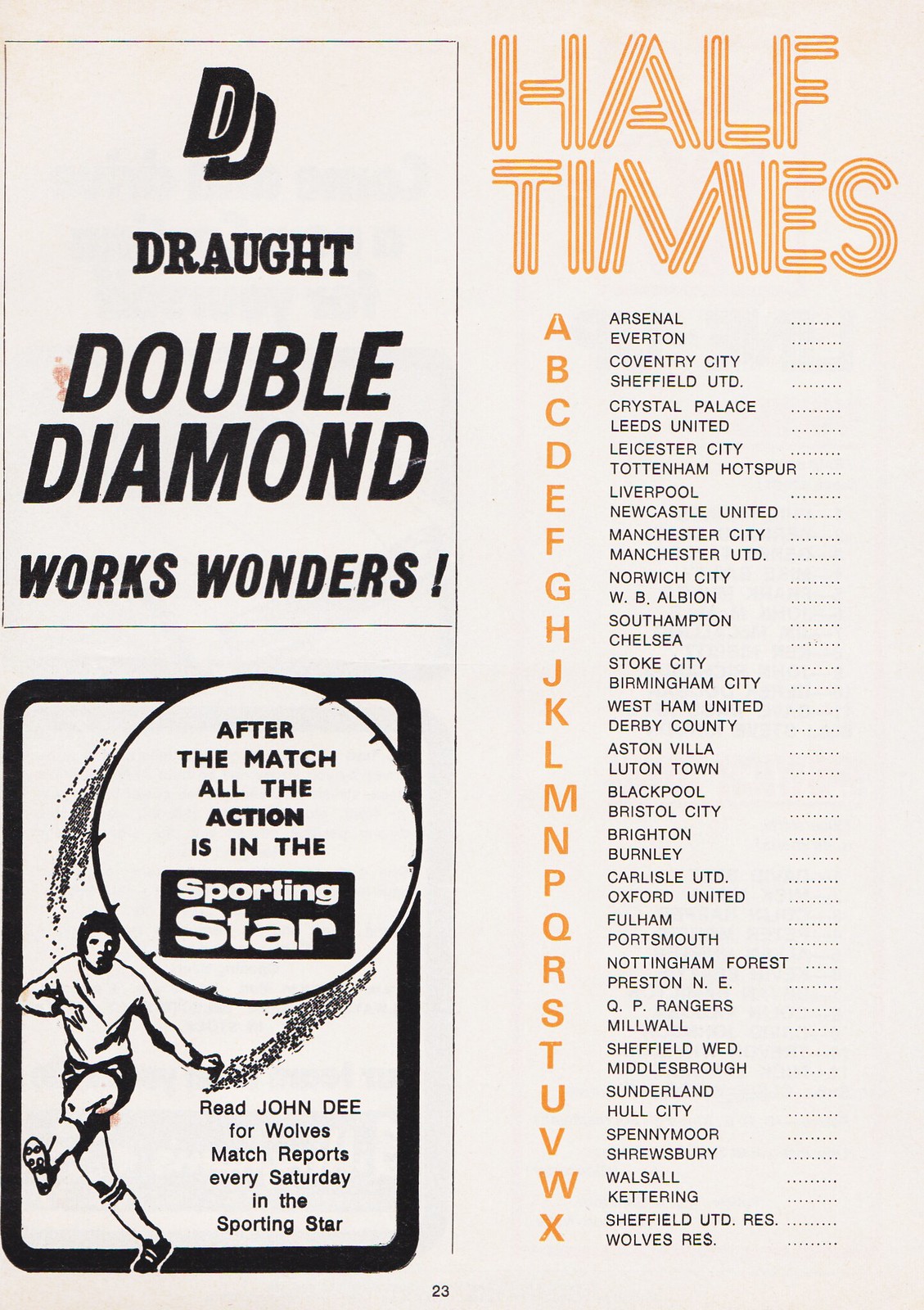The image is a page from a sports magazine prominently featuring football (soccer) content. On the top left, there is an ad for a beverage reading "Didi Draught Double Diamond Works Wonders!" Below this is another advertisement depicting a soccer player in action, kicking the ball while wearing a soccer outfit. Above the player is a white circle outlined in black with the phrase: "After the match, all the action is in the sporting star." Further description in the ad promotes, "Read John Dee for Wolves match reports every Saturday in the Sporting Star."

On the top right of the image, the title "Half Times" is displayed. Below this title, a comprehensive list of football teams and their matchups is arranged alphabetically, from A to X. The list includes:

- A: Arsenal vs. Everton
- B: Coventry City vs. Sheffield United
- C: Crystal Palace vs. Leeds United
- D: Leicester City vs. Tottenham Hotspur
- E: Liverpool vs. Newcastle United
- F: Manchester City vs. Manchester United
- G: Norwich City vs. West Bromwich Albion
- H: Southampton vs. Chelsea
- J: Stoke City vs. Birmingham City
- K: West Ham United vs. Derby County
- L: Aston Villa vs. Luton Town
- M: Blackpool vs. Bristol City
- N: Brighton vs. Burnley
- P: Carlisle United vs. Oxford United
- Q: Fulham vs. Portsmouth
- R: Nottingham Forest vs. Preston North End
- S: Queens Park Rangers vs. Millwall
- T: Sheffield Wednesday vs. Middlesbrough
- U: Sunderland vs. Hull City
- V: Plymouth vs. Shrewsbury
- W: Walsall vs. Kettering
- X: Sheffield United Reserves vs. Wolves Reserves.

The image effectively combines advertisements and detailed match schedules, reflecting a typical layout of a sports magazine page focusing on English football clubs.